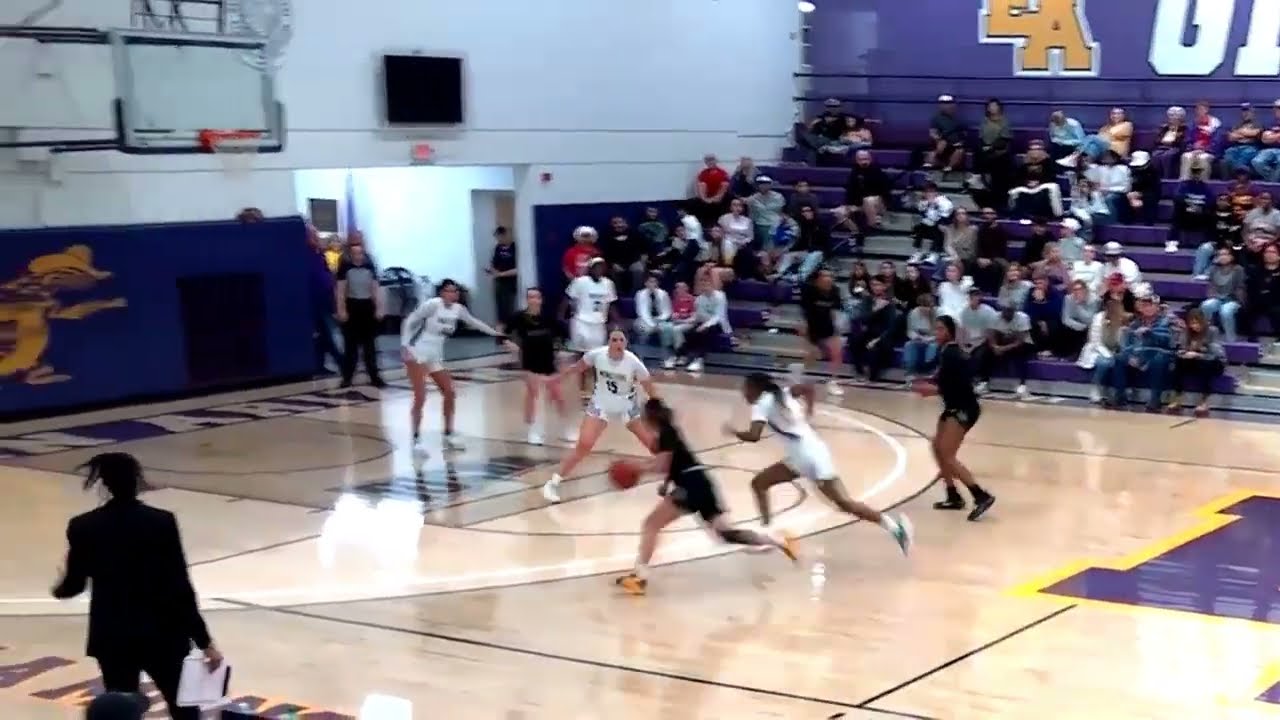The blurry photograph captures an intense moment during a likely high school girls' basketball game set indoors. The image shows two teams: one in black jerseys and shorts, the other in white. The team in black currently has possession of the ball, with a player charging down the court towards the hoop, while a defender in white braces herself at the free throw line. The game unfolds in front of a packed crowd seated on purple bleachers situated in the top-right of the frame. Visible above the spectators are partially obscured letters, "EA... O", hinting at the gymnasium's name. The background features white walls and a stretch of purple padding at the baseline, which includes a yellow mascot that is indistinct but possibly a duck wearing a cowboy hat. In the bottom left, a woman, possibly the coach, stands with her back to the camera, clad in a formal black suit and holding a white clipboard, attentively watching the action unfold on the court.